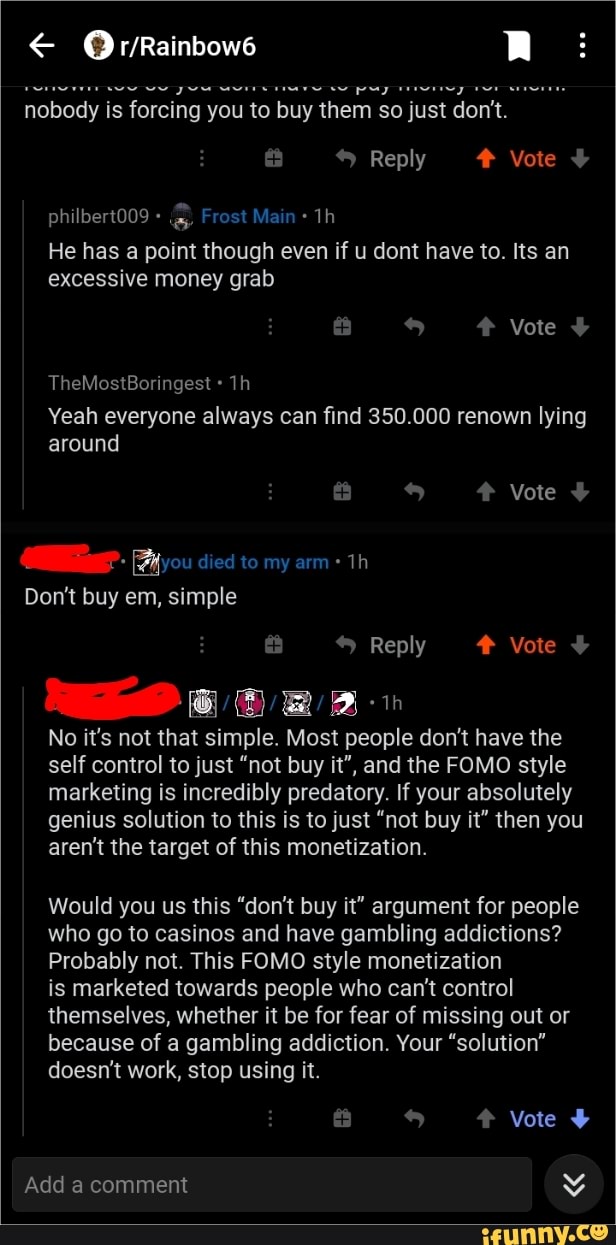This image is a screenshot taken from a mobile phone, depicting a conversation on the Reddit community r/rainbow6. At the top of the screen, there is a back arrow on the left, followed by a small circular profile icon. The title 'r/rainbow6' appears next, with a bookmark icon and three vertical dots for more options situated on the right-hand side.

Below the title, part of a comment is visible, reading: "Nobody is forcing you to buy them so just don't." The portion above this comment is partially cut off. Underneath the comment, there are options to reply and vote, indicated by a left arrow and the word 'vote,' respectively. The vote option is highlighted in red. Further down, the name 'PhilbertT009' appears, followed by his comment: "Frostman. He has a point though even if you don't have to. It's an excessive money grab."

The image includes additional conversation threads, with some messages partially obscured or scratched out. One such message simply states, "don't buy them simple," but both the preceding profile information and the name are obscured. Near this message, four profile icons are visible, followed by two paragraphs of text.

The overall image conveys users' discussions and opinions on the topic of in-game purchases, highlighting a critique of what is perceived as excessive monetization.